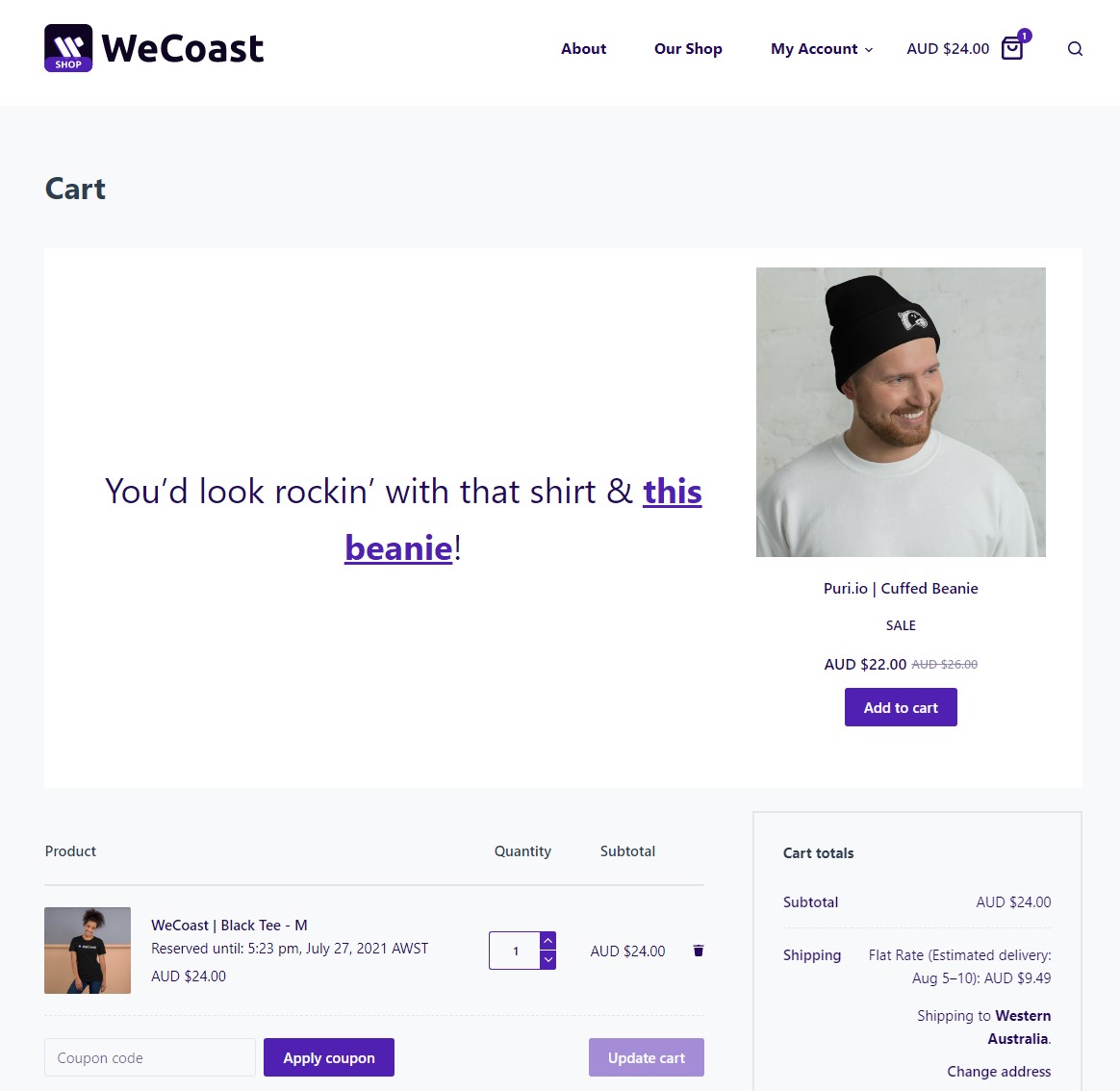In the upper left corner, the website features the "WeCoast" logo, with both the 'W' and 'C' capitalized and displayed in black text. Adjacent to it on the left side, there are navigation options: "Shop" on a square icon, "About Our Shop," "My Account" which has a drop-down menu, and an icon showing a shopping bag containing one item, with the text "AUD $24" next to it. A search icon is visible as well.

Below this navigation bar, there's another section starting with the word "Cart" on the left. Further down, there's a promotional message that reads, "You'd look rocking with that shirt and this beanie." The word "this beanie" is underlined and in purple. An image to the right displays a white man wearing a black beanie and a white shirt, looking to the right. Beneath the image, there is a description: "Puri.io Cuffed Beanie - Sale: AUD $22 (previously AUD $26, which is crossed out in gray)." An "Add to Cart" button in purple with white font is positioned below this description.

Next, there's a section titled "Product" that lists "WeCoast Black Tee - Reserved until 5:23 PM, July 27, 2021 AWST." Alongside this text, there's a photo of a woman wearing a black t-shirt. The product information notes a quantity of one and a subtotal of "AUD $24." Also present is a small trash can icon for removing the item.

At the bottom left of the section, there's a "Coupon Code" field for entering discount codes, accompanied by an "Apply Code" button.